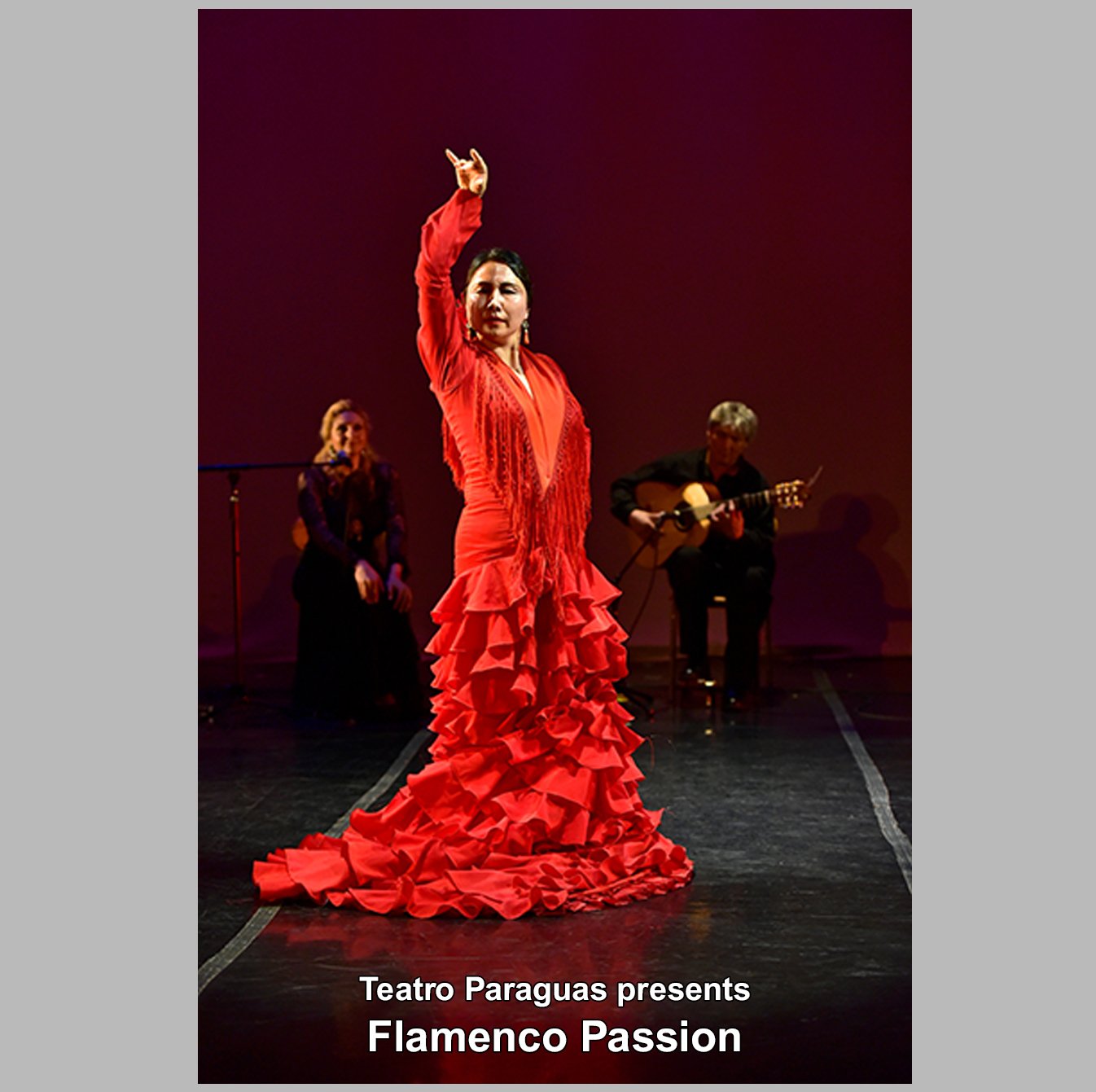In this dramatic stage photograph, the central figure is a captivating flamenco dancer, striking a poised stance with one arm gracefully raised and fingers elegantly pointed. She is adorned in a stunning, full-length, flowy red dress that cascades to the floor and features intricately ruffled layers at the bottom. Her look is completed with dangling earrings that catch the light. The stage is dimly lit, drawing focused attention to her commanding presence.

In the background, partially shrouded in darkness, are two musicians providing accompaniment to her passionate performance. On one side is a blonde woman seated behind a microphone, likely serving as the backup vocalist, dressed in a black gown. Opposite her, a blonde man clad in a black shirt and trousers is captured strumming a Spanish guitar. Both are integral to the enchanting atmosphere of the performance. At the bottom of the picture, a text reads, "Teatro Paraguas presents Flamenco Passion," hinting that this evocative display takes place in Paraguay. The dark, possibly tiled or concrete stage floor further enhances the intensity of the scene.